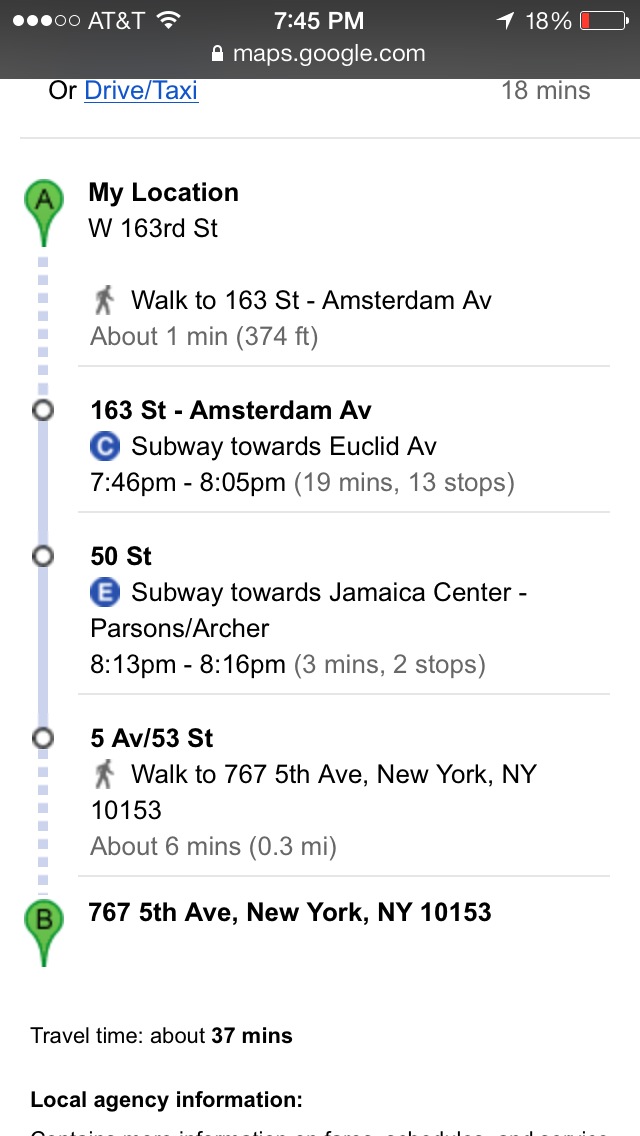This image is a detailed screenshot of Google Maps directions on an AT&T phone at 7:45 PM with only 18% battery life, indicated by a red battery icon, and logged into maps.google.com. The starting location is W163rd Street, where the user needs to walk to W163rd Street and Amsterdam Avenue, approximately 1 minute or 374 feet away. From there, they should take the subway (C line in a blue circle) towards Euclid Avenue at 7:46 PM. This journey lasts 19 minutes over 13 stops, ending at 8:05 PM. Next, they need to transfer at 50th Street to the E line towards Jamaica Center, Parsons Archer, leaving at 8:13 PM and arriving in 3 minutes after 2 stops at 8:16 PM. The final leg involves walking to 767 5th Avenue, New York, NY 10153, which takes about 6 minutes over a distance of 0.3 miles. The total estimated travel time for this route is approximately 37 minutes.